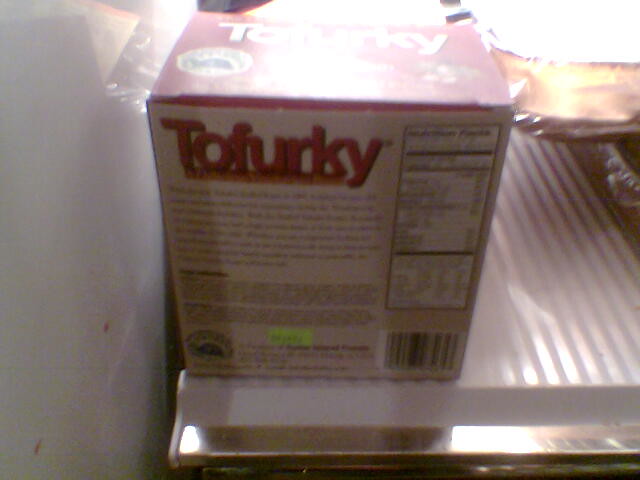This photograph, taken from inside a refrigerator, focuses on the back of a Tofurky box. The box is prominently positioned on a white plastic shelf, above what appears to be a produce drawer indicated by a silver or gold handle. The top of the Tofurky box is red with "TOFURKY" written in bold white letters. The back of the box is white and features nutritional information, although the text is not clearly legible due to the image’s graininess and blurriness. There are also some other objects in the fridge, including something wrapped in foil in the upper left corner, but they are not distinctly visible. The scene is lit from behind, highlighting minor stains and food particles on the refrigerator walls. A bright green price tag on the Tofurky box is partially visible, though its text remains unclear. The overall composition emphasizes the Tofurky box against the somewhat cluttered backdrop of the refrigerator interior.